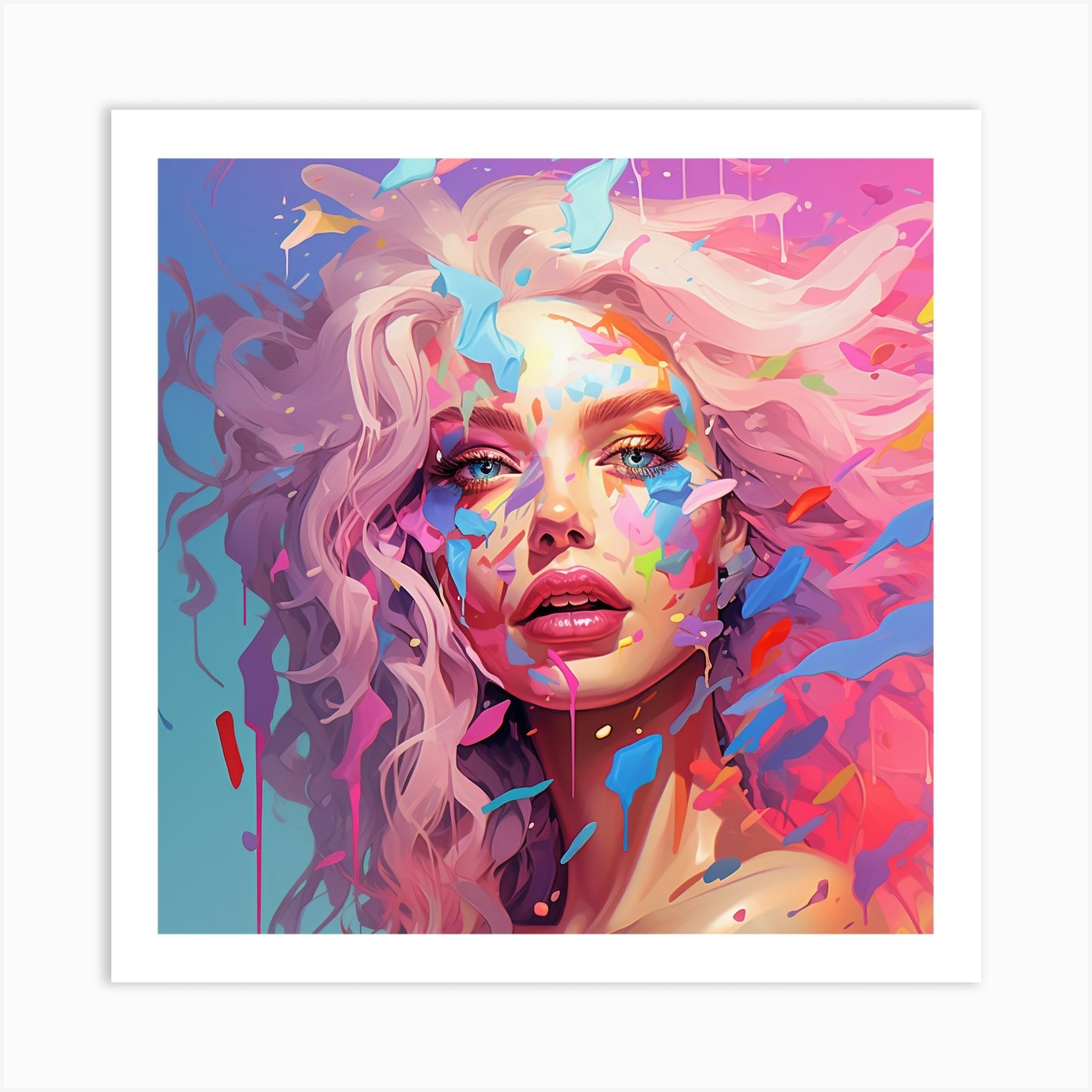The image is a detailed piece of abstract artwork featuring a young woman, likely in her early 20s, displayed within a white picture frame mounted on a white wall. The artwork itself is bordered by a gray outer edge. The woman, who is depicted from the top of her head down to about her shoulders, has light, whitish-blonde hair that fans out towards the upper right corner and cascades down to the bottom left of the picture. Her complexion is fair, and her striking blue eyes are accentuated with manicured brownish eyebrows and prominent eyelashes coated in mascara. She wears vivid, bright pink lipstick, with her mouth slightly open to reveal her top teeth.

The painting's background is divided into two primary colors: pink on the right and blue on the left, fading into a gradient at the top. Her hair color has a hint of lavender, adding to the abstract nature of the portrait. The woman’s image is surrounded and overlaid by dynamic brush strokes and splotches of various colors, including blue, red, yellow, and purple, some of which seem to float in midair, creating a vibrant, energetic composition.